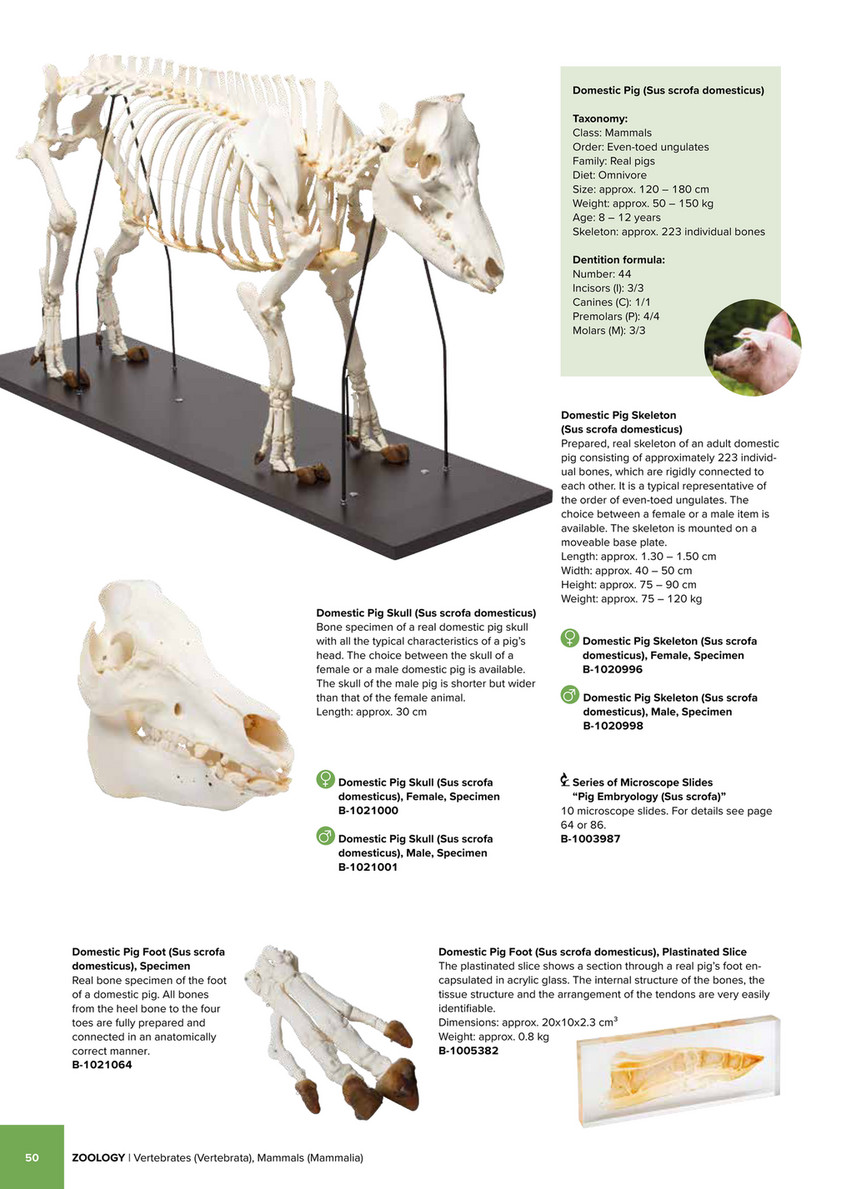The image displays a detailed model of a domestic pig's skeleton, mounted on a board with metal posts as if in a museum exhibit. The skeleton is accompanied by various pieces of text providing extensive information about the anatomy and dimensions of the pig, all set against a white background. To the right of the skeleton model, there are smaller images, including a close-up of a pig's pink head and detailed shots of the snout and a hoof. These images are supplemented with several boxes of text giving further detailed information about the domestic pig. At the bottom of the image, the source is credited to zoology.